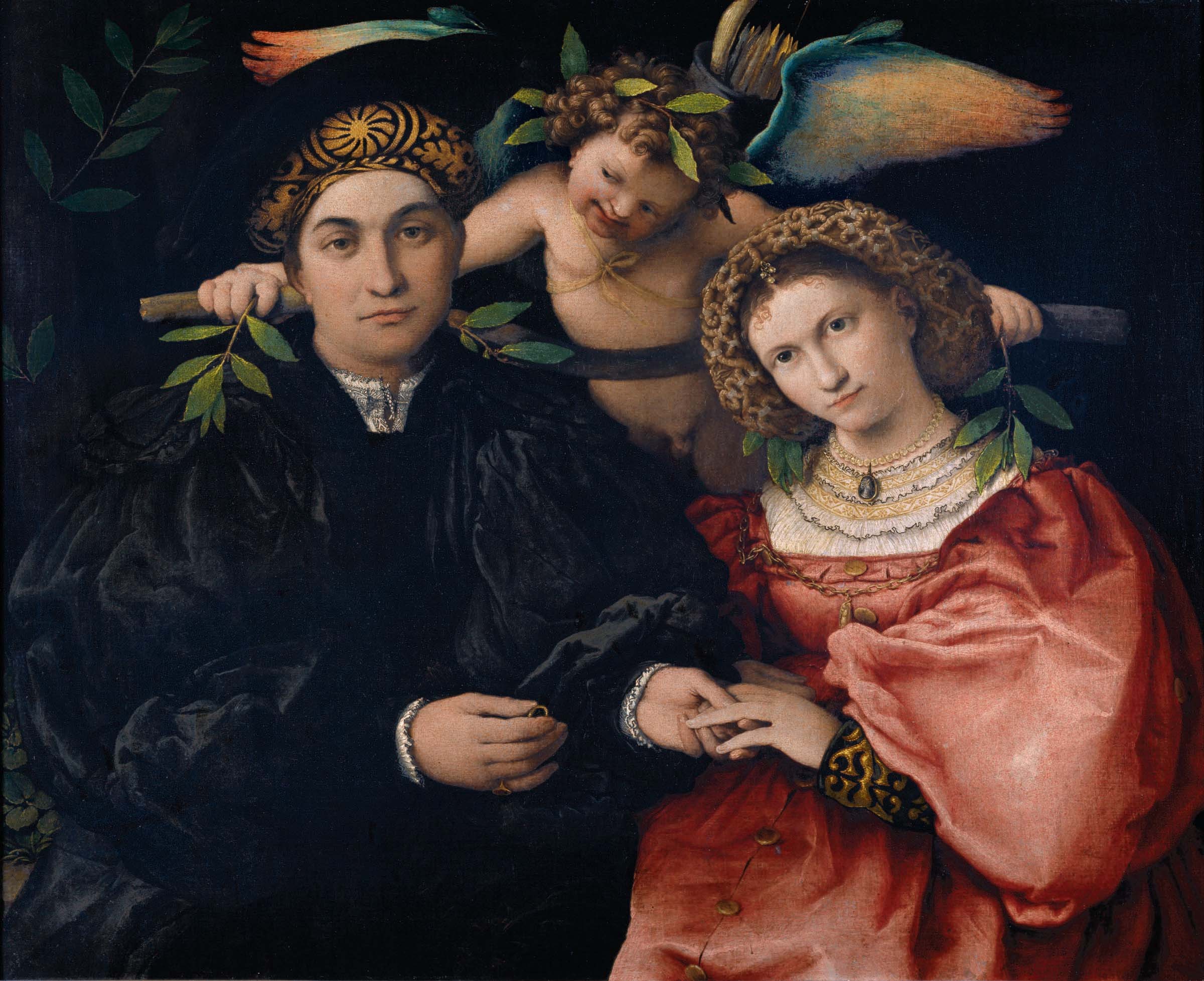The painting depicts a classical scene, likely from the Renaissance or Victorian era, featuring three figures. On the left stands a man dressed in a long black robe with poofy sleeves and a black helmet adorned with gold trimming. He holds a ring in his right hand and the left hand of a woman beside him. The woman, positioned on the right, is adorned in a dark red gown with large, poofy sleeves. Her hair is pulled back in an embellished, bedazzled hairnet, and she is decorated with multiple necklaces of gold, silver, and pearls, along with a black brooch. She has her left hand in the man's hand, anticipating the placement of the ring. Above and slightly behind them floats a cherubic figure, a small curly-haired angel or cupid with wings and leaves in its hair. The angel reaches down with leaves towards the man's shoulders, adding an ethereal touch to this intricate and emotive scene.